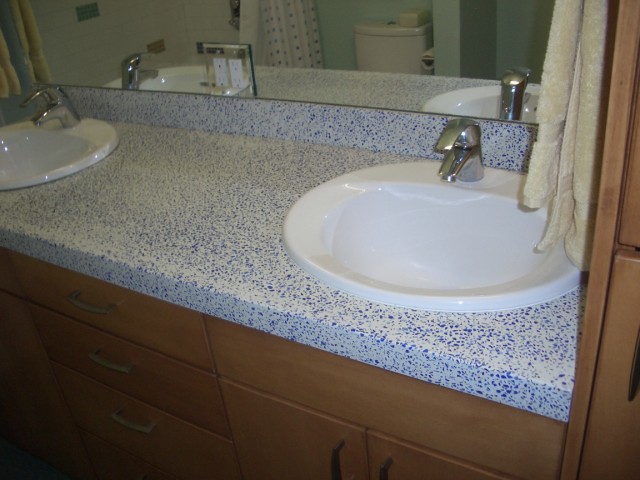The image depicts a detailed view of a modern bathroom, focusing on a double sink countertop. The countertop is crafted from granite, featuring a white base interspersed with blue and gray speckles. Each sink is made of pristine white porcelain, complemented by sleek silver faucets. Behind the sinks, a large mirror spans the width of the countertop, incorporating two built-in outlets with mirrored borders for a seamless appearance. Below the countertop, light brown cabinets and drawers provide ample storage space, contributing to the bathroom's elegant and functional design.